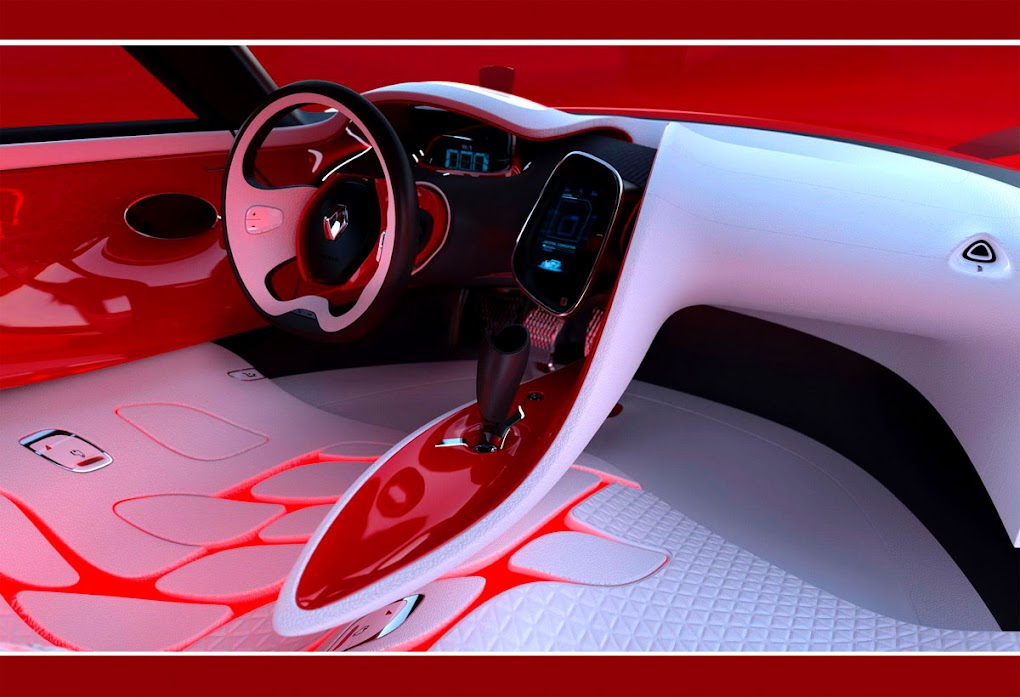This image appears to show the interior of an unconventional vehicle, possibly a futuristic or concept car. The overall color scheme is dominated by red, white, and black. The distinctive feature is a red center console with a black gear shifter positioned in a pointed, oblong shape. The dashboard is mostly smooth and white, adorned with lights and gauges, contrasted by a black section and a vibrant red background. The steering wheel has a unique design with a white body, a black center, and red elements. Notable also are the unconventional seating areas, which seem curved and lack traditional backrests. The floor is white with a pattern of red designs, and there is an object resembling a phone on what seems to be the driver's seat. The driver's side door is strikingly cherry red, and there's a handle or component which could indicate a door mechanism. Despite some ambiguity about the nature of the vehicle, the lack of pedals and the stylized interior suggest it might be a conceptual or rendered vehicle environment.